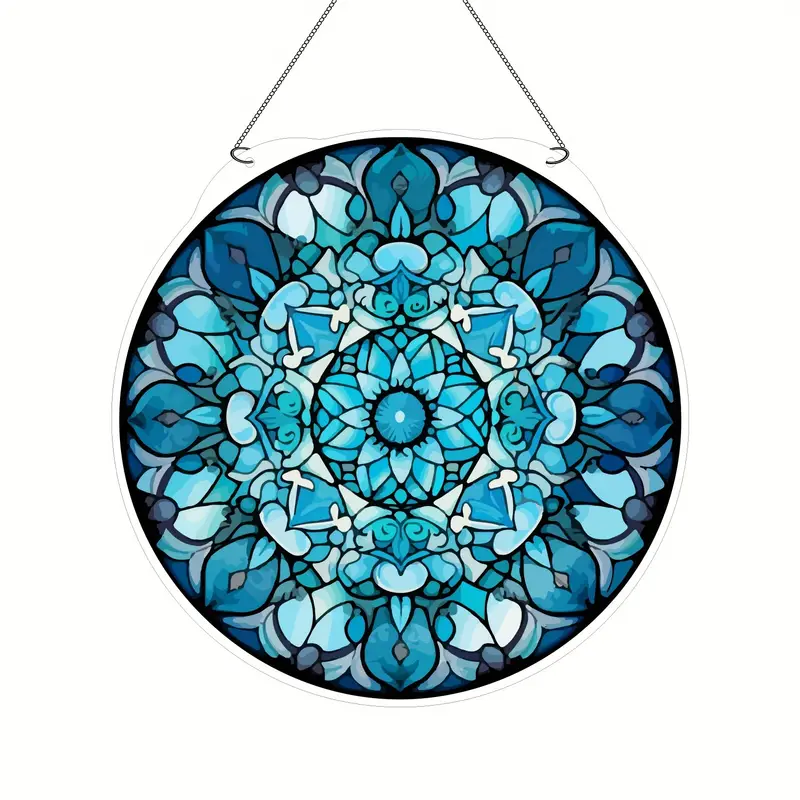The image features a hanging ornament, likely made of glass, painted in varying shades of blue. The ornament is suspended by two metal chains. At its core, there is a white circle bordered by a black ring, emanating tentacle-like rays resembling the sun. Surrounding this central motif is a teal section followed by a larger pattern of circular layers. These layers consist of flower petal designs in light blue hues, from teal and aqua to sky blue. The next prominent feature is a black circle encompassing triangular and rounded heart-like shapes with flat bottoms, contributing to the ornate design. The outermost layer displays an intricate floral pattern in different shades of sky blue, complemented by further detailed blue and white designs along the perimeter. The entire composition showcases a harmonious blend of shapes and colors that enhance the elegance of the ornament.